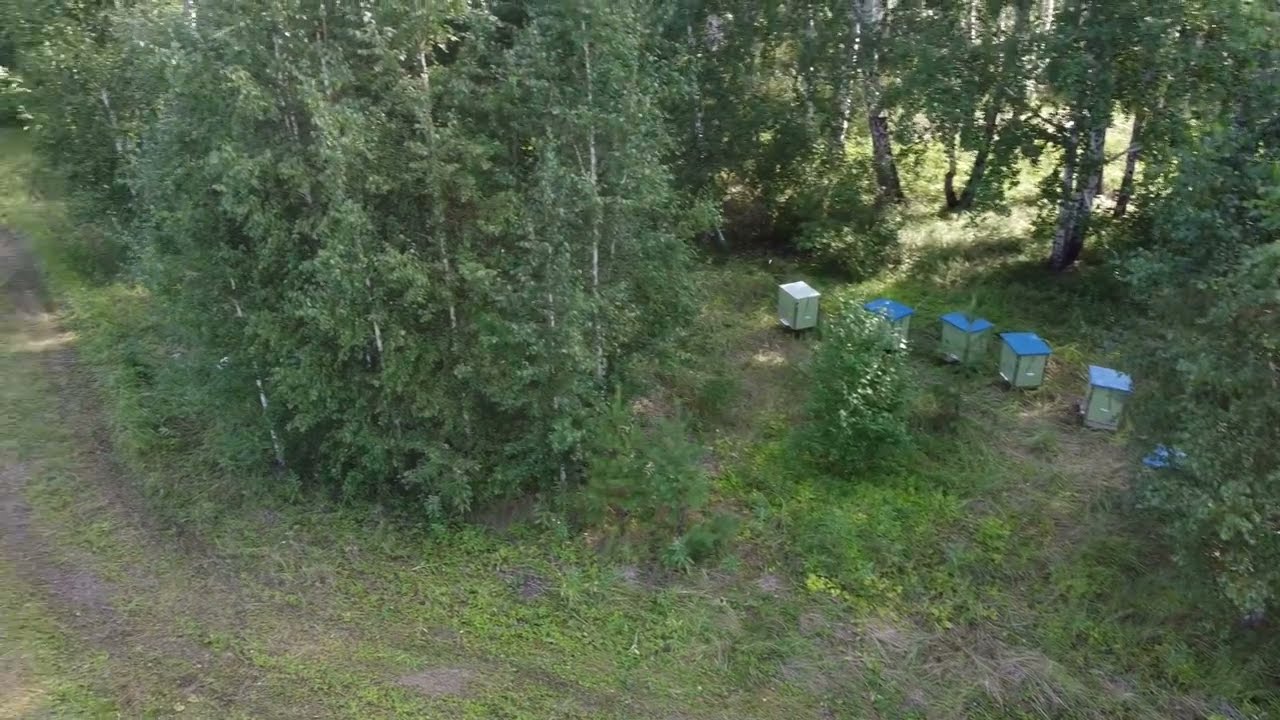The image captures a sunny day in a wooded area as seen from an elevated viewpoint, revealing a small clearing with five glass-sided boxes lined up. Four of the boxes have blue roofs, while the one on the far left has a white roof. These box-like structures, approximately two feet tall, are arranged in a line in front of a single bush. In the left-hand bottom corner, there are dirt tracks made by vehicles, with patches of grass growing in between. The rest of the image features lush green trees, and sunlight filters through the forest canopy, illuminating the scene and highlighting the dense foliage beyond the clearing.